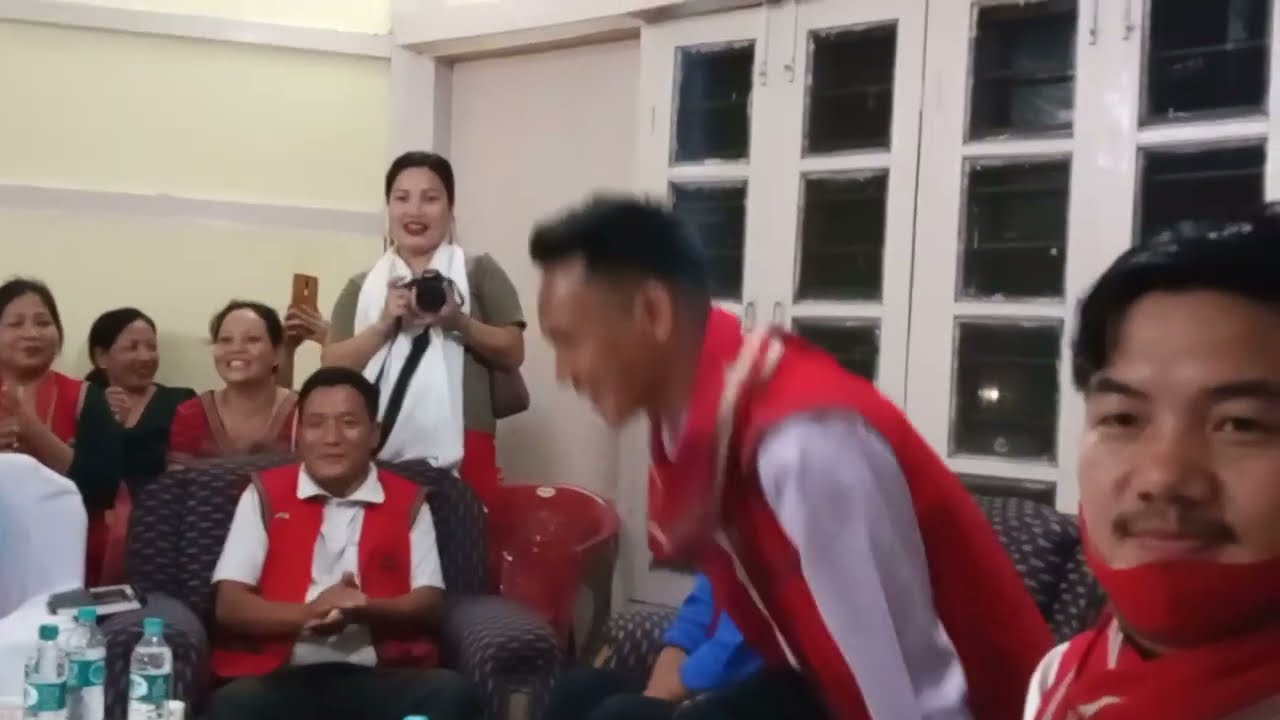The photo is an indoor celebration capturing a moment of joy and camaraderie among seven individuals, four women, and three men, predominantly of Asian descent. They are gathered in a room featuring white-panelled walls and windows with white woodwork. The walls are a greenish-yellow hue, and the group is seated on armchairs with dark navy-blue and patterned upholstery. In the center, a man wearing a white shirt and red vest appears blurry as he stands mid-motion from his chair, smiling. To his right, another gentleman, young with black hair and a slight mustache, also in a white shirt and red vest, sits on a black-and-grey upholstered couch, wearing a red scarf-like accessory around his neck. 

Next to him, faintly visible are the arms and blue pants of another person seated on the couch. On the left side of the man in motion, a middle-aged man claps his hands joyfully, dressed similarly in a white shirt, red vest, and black pants. 

Behind him, a woman in a green shirt with a white scarf draped over her shoulder can be seen holding a camera, smiling with maroon makeup visible. To her side, another woman in a red dress, also smiling, sits and enjoys the moment. Next to her, to the left edge of the image, sits another woman in a black dress, also smiling and looking towards the others. Partially cut off by the left side of the frame is the final woman, dressed similarly in a red dress and clapping. 

In the foreground, on the lower left, three bottles of water rest on a small surface. The joyous atmosphere is palpable, with everyone either smiling, clapping, or capturing the special moments with their cameras.